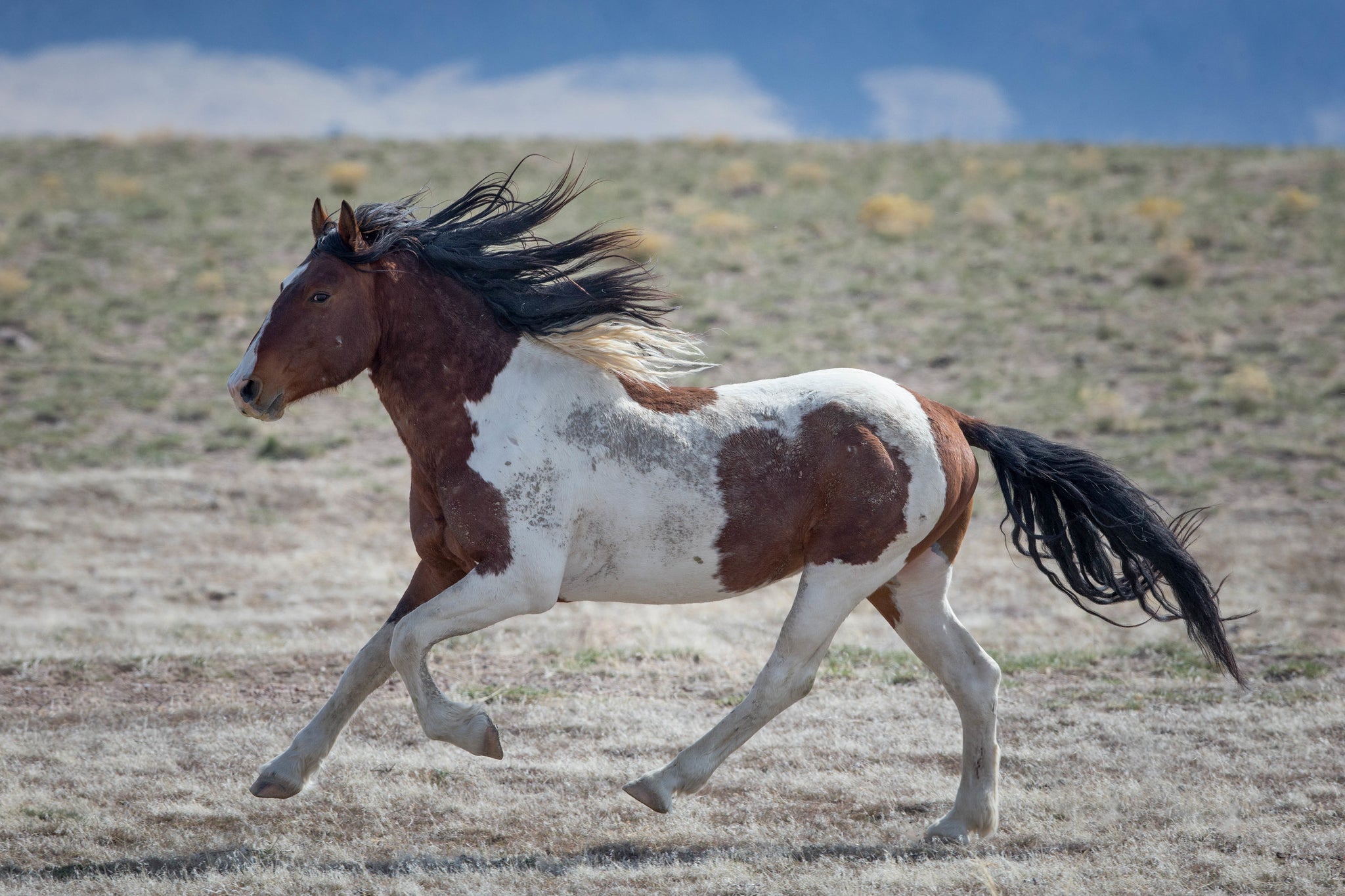The image captures a striking scene of a wild horse in mid-trot across the barren grasslands of the American West. The open plain, dotted with sparse, dead grass and bushes, stretches under a beautiful blue sky with wispy white clouds. The horse, a pinto with a combination of brown, white, and some gray spots, exhibits signs of wear and tear with visible scars on its head and body, hinting at its rugged life in the wild. Its mane and tail are primarily black, accented with some blonde at the bottom quarter of the mane. The horse's expressive eyes seem to gaze toward the camera, adding a sense of connection with the viewer. Despite the somewhat blurry background, the horse's dynamic motion is vividly captured, with its mane and tail flowing dramatically in the wind. The scene is a vivid snapshot of the untamed natural beauty and raw vitality of wild horses.